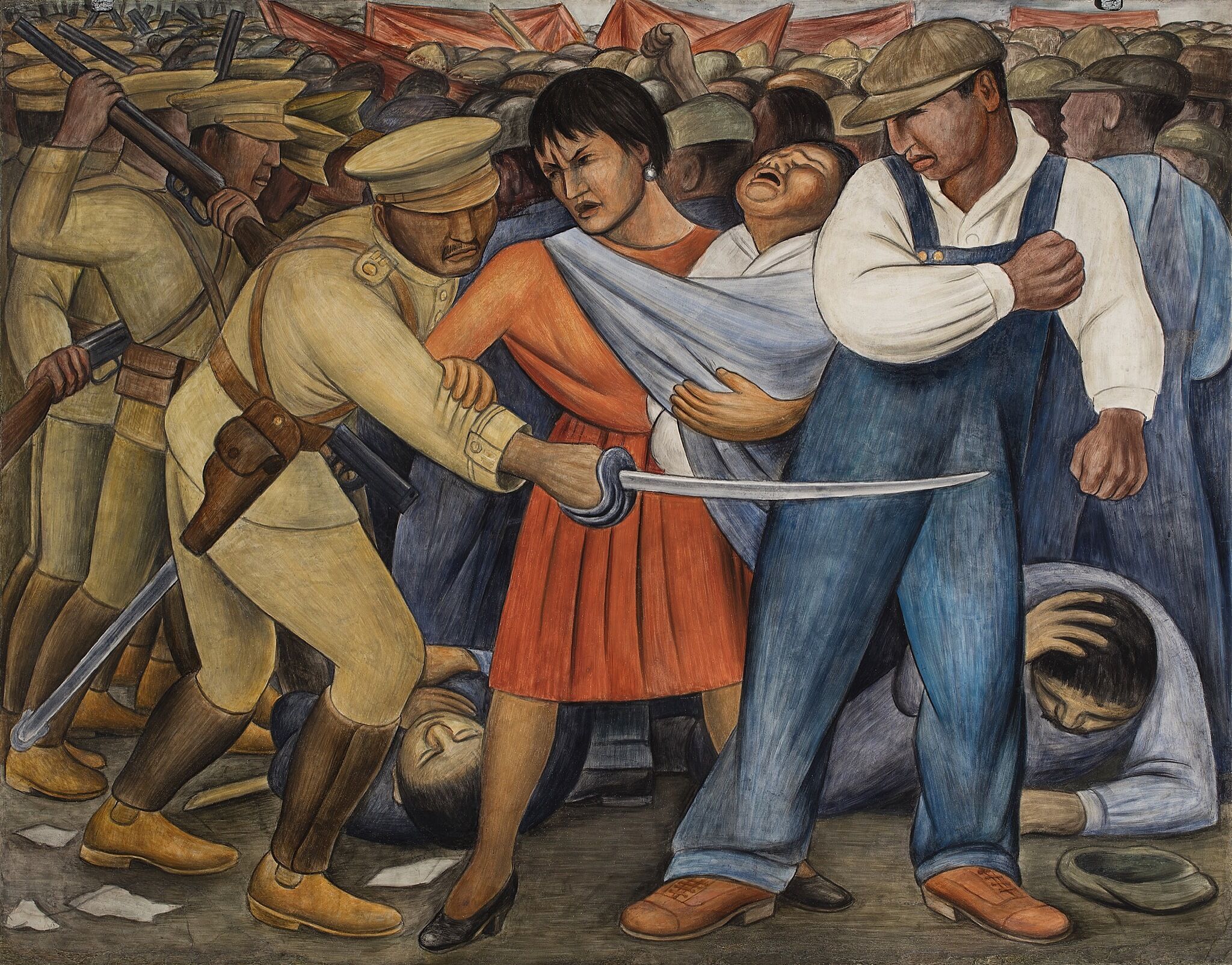This is an intricately detailed artistic drawing depicting a chaotic and violent scene likely set in an earlier time. The foreground prominently features several figures in distress amidst a brutal confrontation. On the left side, a group of soldiers wearing tan colored hats and outfits with brown boots are seen imposing force. One soldier, centrally positioned, aggressively thrusts a sword towards the right, aiming at a defiant woman in an orange dress who clutches a baby in her arms with an expression of furious defiance. Next to her, a man dressed in a white long-sleeve shirt, a blue denim jumper, and brown shoes, under a tan hat, recoils in fear, pulling his arm back.

In the background, more soldiers appear, some brandishing rifles poised to strike. The overall atmosphere suggests a widespread sense of victimization, with heads of numerous people visible, appearing as a sea of oppressed individuals. On the lower right, a man is depicted on the ground, shielding his head with an arm, suggesting he has been beaten severely. The scene exudes a sense of public oppression, resonating with the historical paintings portraying common citizens subjected to brutal authority, possibly in an Asian context, illustrating the harsh reality of societal unrest and authoritarian violence.